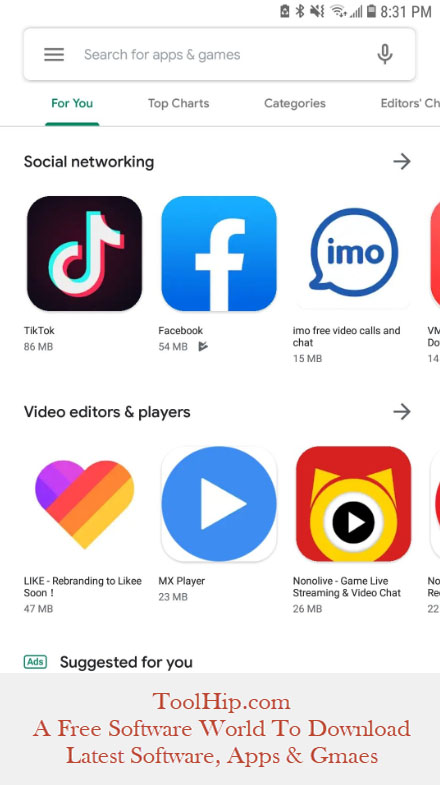The screenshot displays a section of what appears to be a mobile app store interface. 

**Top Bar:**
- At the very top right, there are icons indicating battery level, Bluetooth connectivity, sound settings, Wi-Fi status, and the current time, which is 8:31 PM.
- To the left of these icons, there is a hamburger menu button and a search bar labeled "Search for apps and games."

**Main Section:**
- The screen is segmented into various headers starting with "For You," "Top Charts," and "Categories."
- Below these headers is a section dedicated to "Social Networking" featuring a series of apps with descriptions and details.
- Listed apps under "Social Networking" include:
  - **TikTok**: This app is represented with a square icon and requires 86 megabytes of space.
  - **Facebook**: This app is represented with a right arrow and requires 51 megabytes of space.
  - **IMO**: Labelled with speech bubble icons indicating it is for video calls and chat.

**Video Editors and Players Section:**
- Below the social networking apps, the next header reads "Video Editors and Players."
- Featured apps in this section include:
  - **Zoom**: A widely used video conferencing app.
  - **MX Player**: A multimedia player requiring 23 megabytes.
  - **NoNoLive**: An app for game live streaming, depicted with a cat symbol and a play button.

**Additional Information:**
- At the bottom of the screenshot, there is a section from ToolHip.com offering free software downloads, including apps and games, labeled as "great apps."

This organized layout suggests that users are viewing a curated list of app recommendations, specifically within social networking and video utility categories.